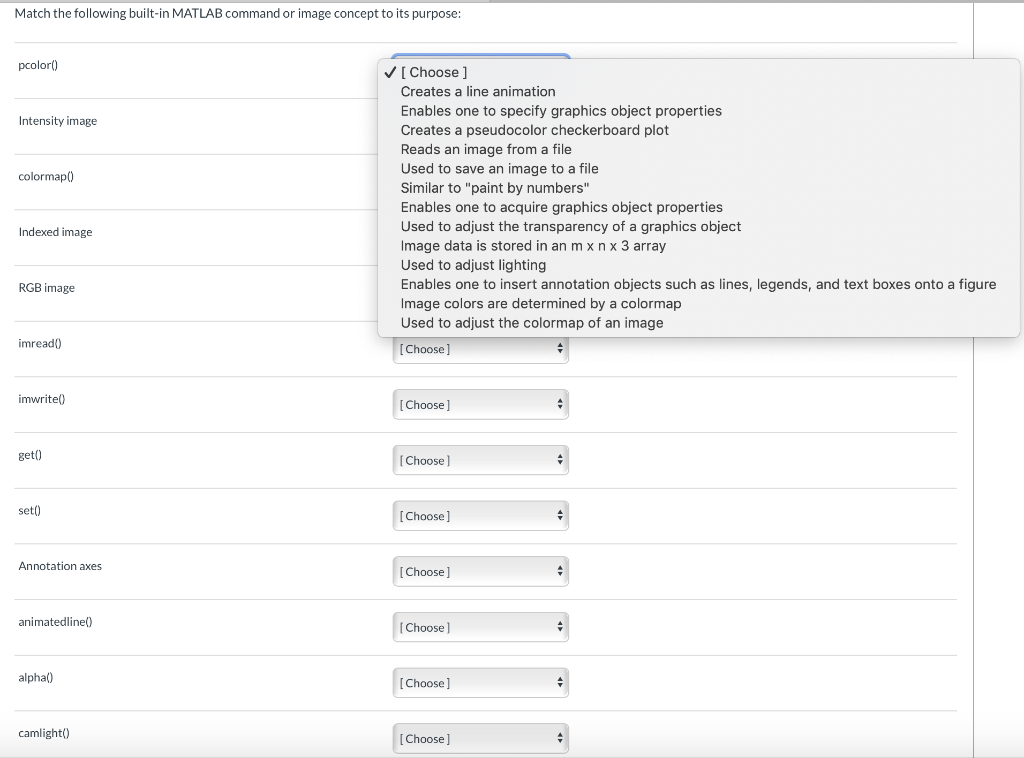In this image, we observe a screenshot set against a pristine white background. The image features very small gray text positioned in the upper left corner with the instruction: "Match the following built-in MATLAB command or image concept to its purpose." Below this instruction, there are faint gray lines separating each section, listing the following terms from top to bottom: PC color, intensity image, color map, indexed image, RGB image, I'm red, I'm right, get, set, annotation axis, animated line, alpha, and cam light.

In the upper right corner of the screenshot, there is a light gray box containing black text, which reads:
- Creates a line animation
- Enables one to specify graphics object properties
- Reads an image from a file
- Used to save an image to a file
- Similar to paint by numbers

The entire arrangement is designed to assist users in matching MATLAB commands or image concepts with their corresponding purposes through visual and textual associations.